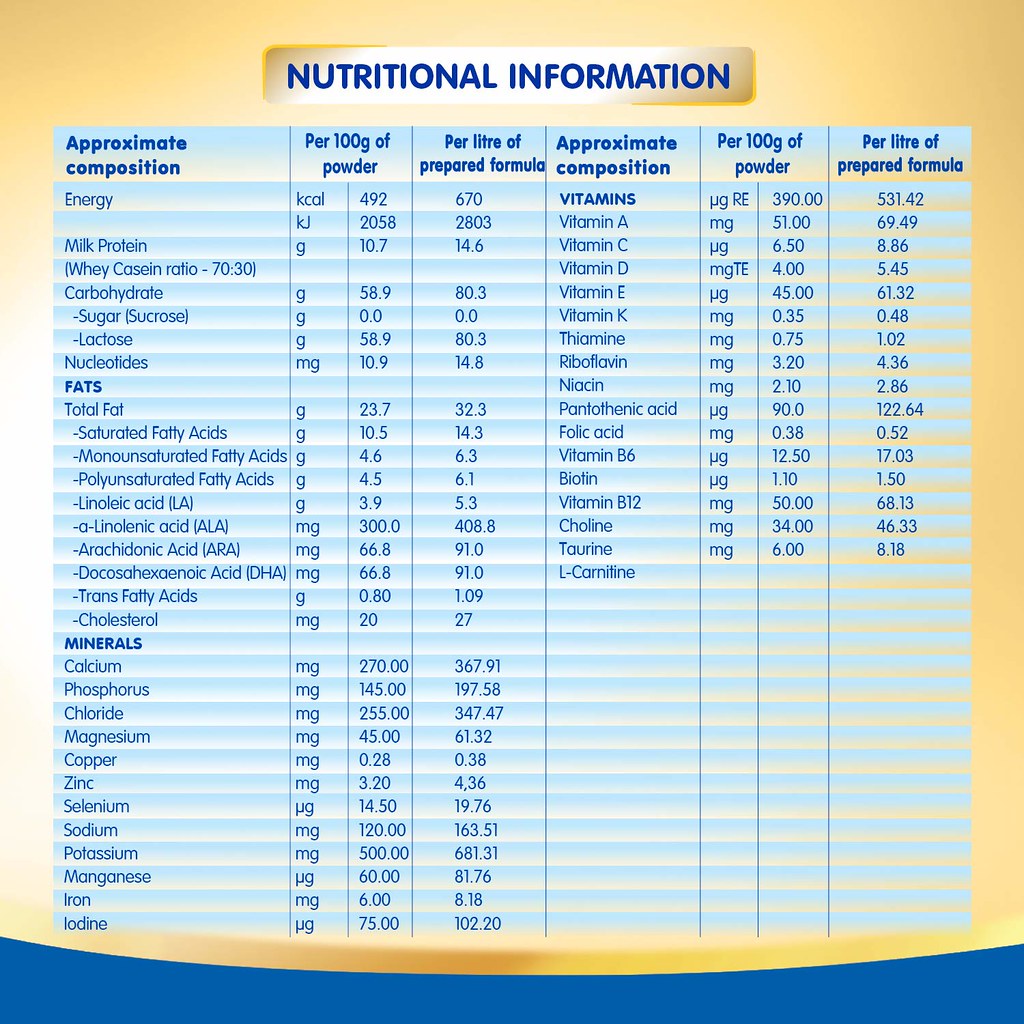The image is a horizontal rectangular sign resembling the back of a baby formula product. The upper half of the background features a golden yellow color that gradually darkens towards the edges, while the bottom half transitions to a deep blue hue. In the middle left, there's a lighter section with a white tone. At the top center, a cream-colored rectangular banner with blue, all-caps text reads "NUTRITIONAL INFORMATION." Below this, a larger blue rectangular section contains detailed nutritional data. 

The information is divided into columns and rows, separated by thin blue lines. The columns are labeled in bold blue font. The headings include "Approximate Composition per 100 grams of powder," "Approximate Composition per liter (L-I-T-R-E) of prepared formula," and then specific nutrient information is presented in a list format. The nutrients listed include energy, milk, protein, sugar, lactose, fats, total fat, minerals, calcium, phosphorus, along with vitamins such as A, C, D, E, and K, and other elements like thiamine, riboflavin, niacin, pantothenic acid, folic acid, vitamin B6, vitamin B12, chlorine, and taurine. The exact quantities for each are provided in corresponding columns for both 100 grams of powder and per liter of prepared formula.